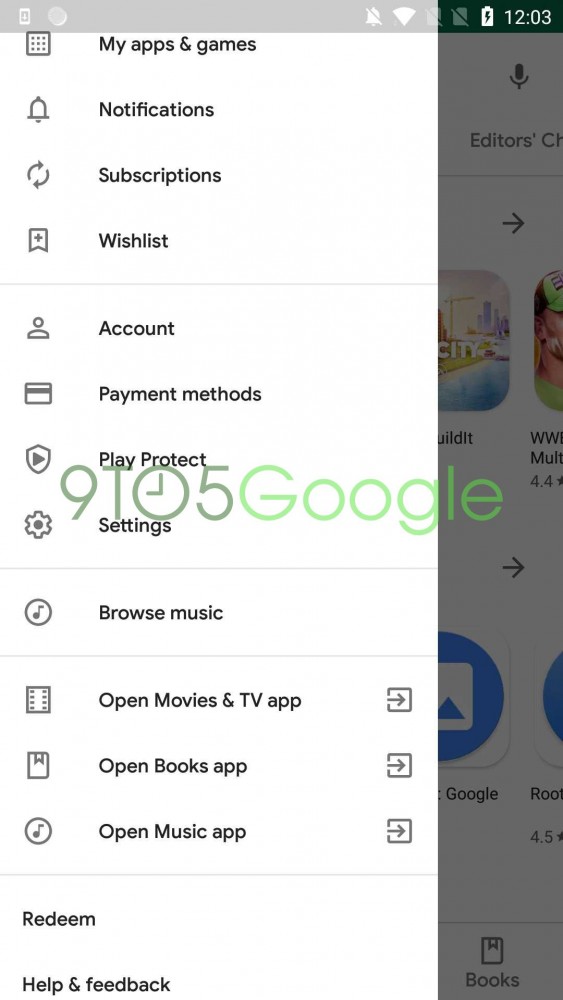Sure, here is a cleaned-up and detailed caption based on the provided information:

---

The top-left corner of the screen displays the phone icon, followed by the location set to Dallas. The status bar shows a full Wi-Fi signal and a fully charged battery with a lightning icon. The time reads 12:03 PM. Below the status bar, various apps and features are present, including notifications, subscriptions, a wishlist, account settings, and payment methods.

Scrolling down, there's an option to 'Pay Per Check,' a '9-5 Google' icon, and settings for browsing music, movies, and books. There's also an option to open the music app, redeem offers, and link to PayPal.

On the right side of the screen, there's the "Sim City" app icon, situated on a white background. At the bottom right, a blue circular icon can be seen, along with the "Books" app icon in the very bottom-right corner. The layout includes a black and grey column on the far right side, making it an efficient grid categorized from 1 to 13.

---